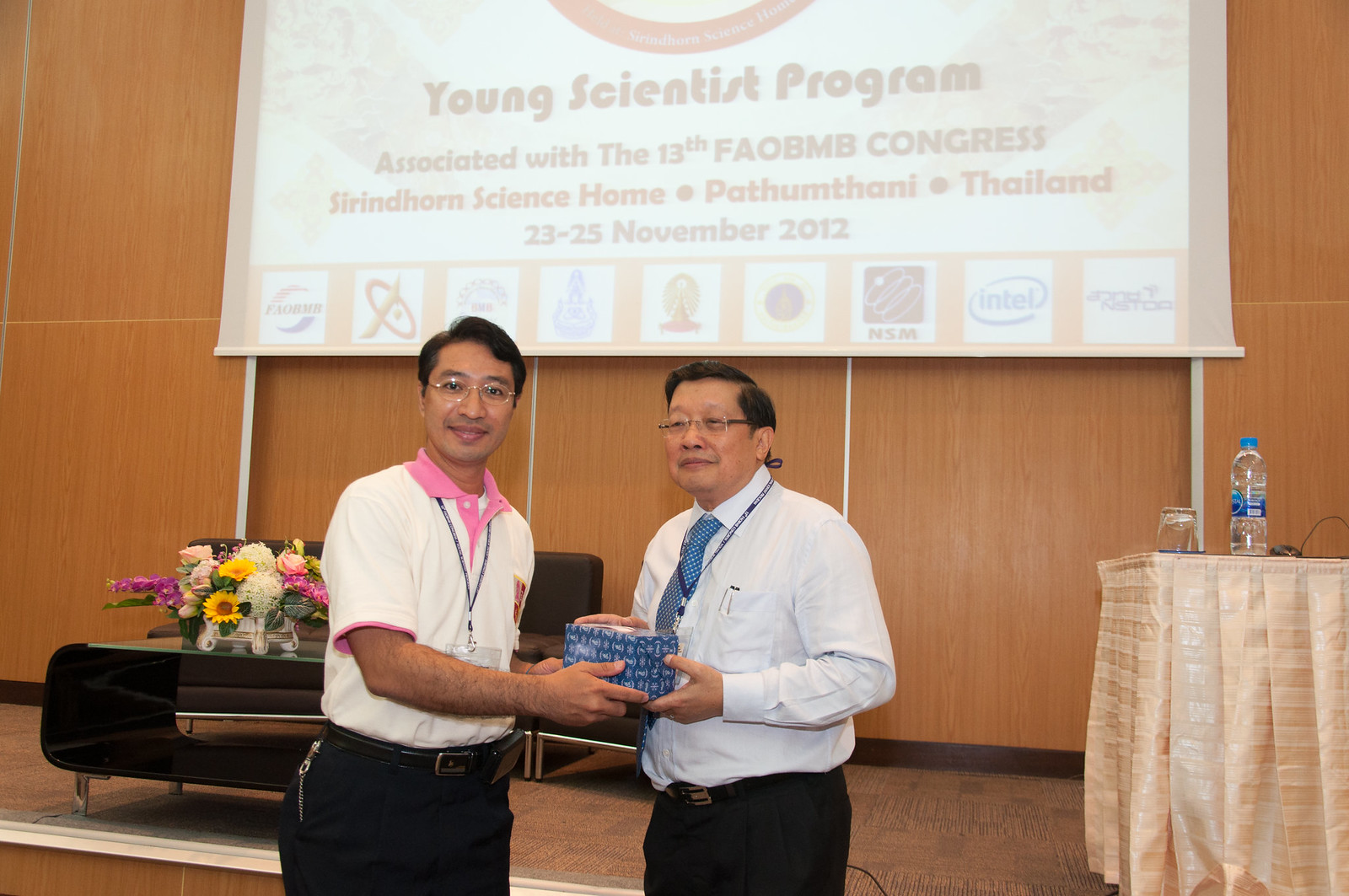In an indoor conference hall, this photographic image captures two Asian men standing beside each other, engaged in the presentation of a box. The man on the left, a younger individual, wears a pink short-sleeve polo shirt paired with a blue lanyard, and glasses. He is presenting a blue and white box to an older, slightly heavier Asian man on the right, who is dressed in a long-sleeve button-up shirt with a blue tie and glasses, with pens tucked into his pocket. Both men are attired in dark slacks and black belts, and are sharing smiles. 

Behind them, a large sign reads "Young Scientist Program, Associated with the 13th FAO BNB Congress, Sirindhorn Science Home, Pathum Thani, Thailand, 23-25 November 2012," partially obscured by a series of logos, including one from Intel. The setting features a table decorated with a bouquet of flowers. Another table to the right holds a bottle of water, indicating a formal presentation environment.